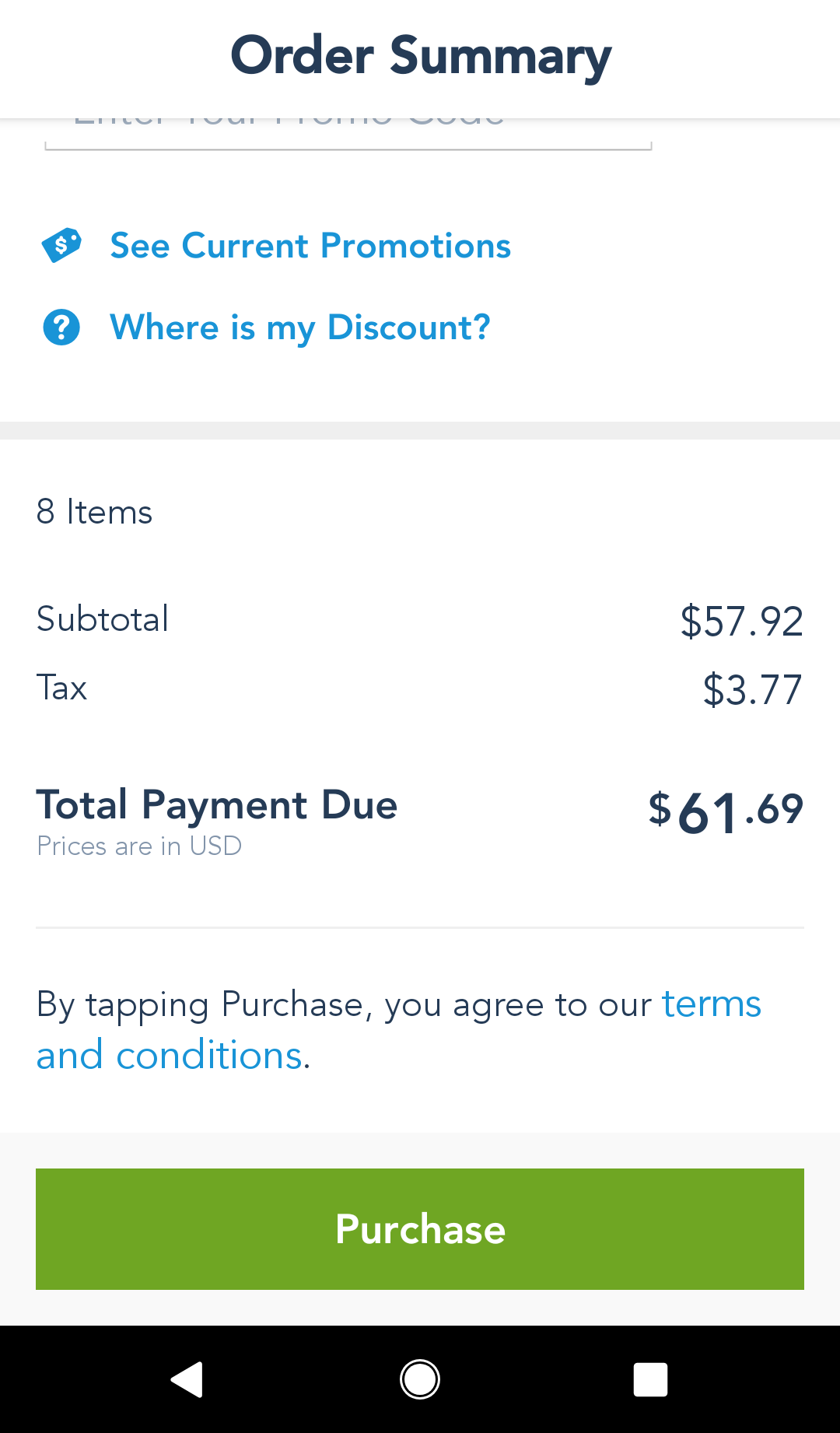**Caption:** 

The image is a detailed view of an Order Summary screen presented on a white background. At the top, the bold black text reading "Order Summary" stands prominently against a white backdrop. Directly below this is a light gray bar, while the "Order Summary" banner seems to be overlaid, revealing some indistinct scrolling information in the background. 

Underneath the banner, there are two blue, clickable texts: "See Current Promotions," accompanied by a sale tag icon, and "Where's My Discount?" displayed next to a blue question mark icon encircled in blue. These options offer further engagement.

Following this, a pale gray thick bar separates the clickable options from the rest of the content. Returning to a white background, the order details are outlined with "Eight Items Subtotal $57.92" and "Tax $3.77" neatly left-aligned for the descriptions and right-aligned for the dollar amounts.

Highlighted in bold and a larger font, the "Total Payment Due $61.69" stands out. Below this total, in small letters, it states that prices are in USD.

A very thin horizontal line separates the totals from a smaller section of text that reads, "By Tapping Purchase You Agree to Our Terms and Conditions." with "Terms and Conditions" colored blue and clickable. 

Another very pale gray bar stretches across the screen, containing a noticeable green button labeled "Purchase" in white letters, ready for user interaction.

Finally, at the bottom of the screen, a black bar features navigational icons: a white left arrow to go back, a central white circle to close, and a white square on the right side. The entire screen is depicted in a vertical, portrait mode layout.